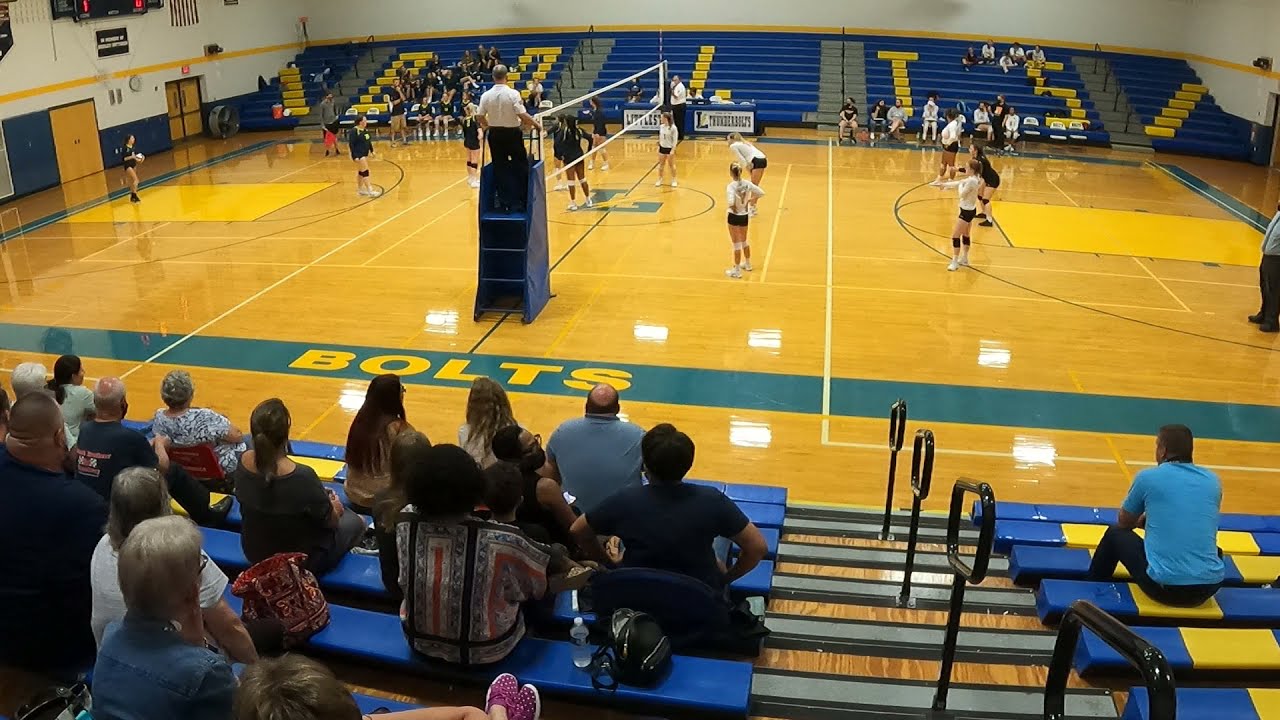The image captures an indoor high school gymnasium during a girls' volleyball game. The bright, shiny wooden floor serves as a combined basketball and volleyball court. On the court, two teams are positioned on either side of the net: one team in white tops with black shorts, and the other team in all black attire. The players in black are preparing to serve. Surrounding the court are blue bleachers with some spectators seated, both near and on the far side. The bleachers are marked with the word "Bolts" in yellow, indicating the school team's name. A referee, dressed in a white shirt and black slacks, stands at the side of the net, while other individuals—likely coaches—are also visible. The left side of the image has a wall with double doors, providing an exit from the gymnasium.